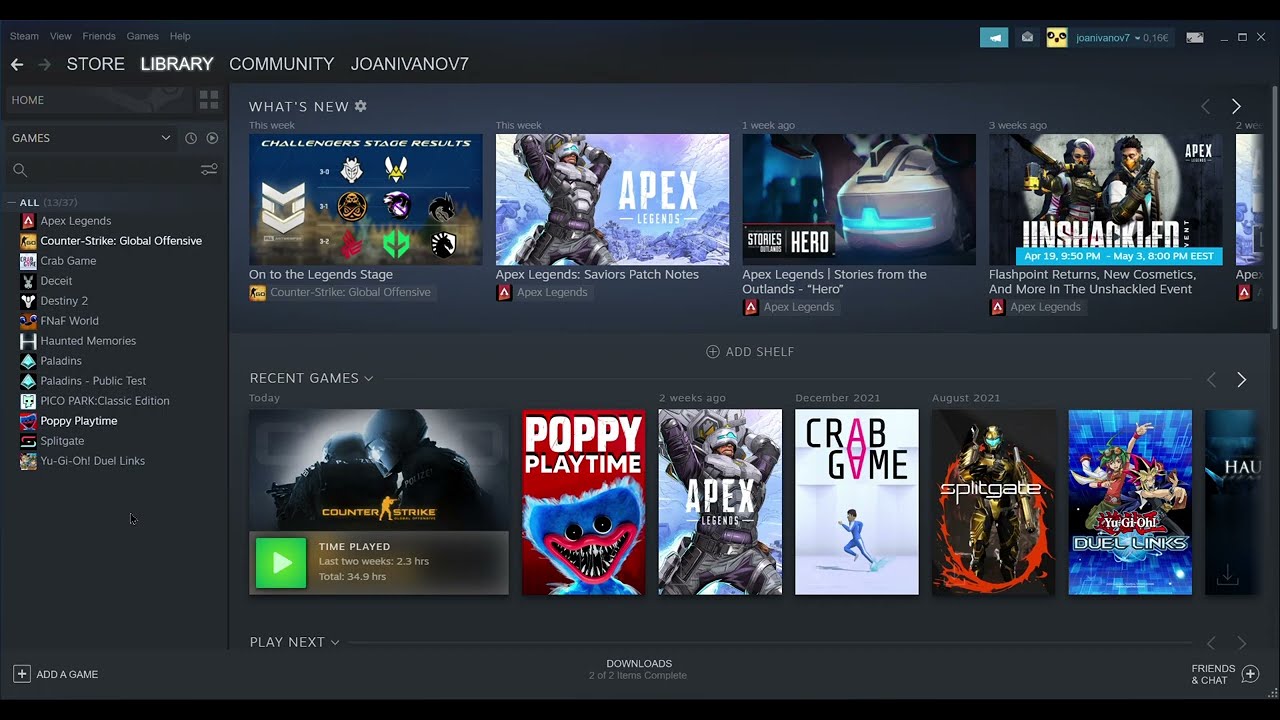The image features a dark grey border with words at the top that are too small to read. Prominently displayed in large white capital letters are the words "STORE," "LIBRARY," and "COMMUNITY," followed by "JOAN IVANOV 7." Positioned to the left below these headings, the words "HOME" and "SAVED" are visible, along with a search box containing a magnifying glass icon. Underneath the search box, the word "ALL" is displayed.

On the main content area, several game titles are listed: "COUNTERSTRIKE: GLOBAL OFFENSIVE," "DESTINY 2," and "PICO PARK." To the right, there's a section labeled "WHAT'S NEW," which features a rotating box of titles, including "APEX," which has a blue background, and "UNSHACKLED," showing two characters with guns. Below this, another section titled "GAMES" lists "POPPY PLAYTIME," "CRAB GAME," and "APEX."